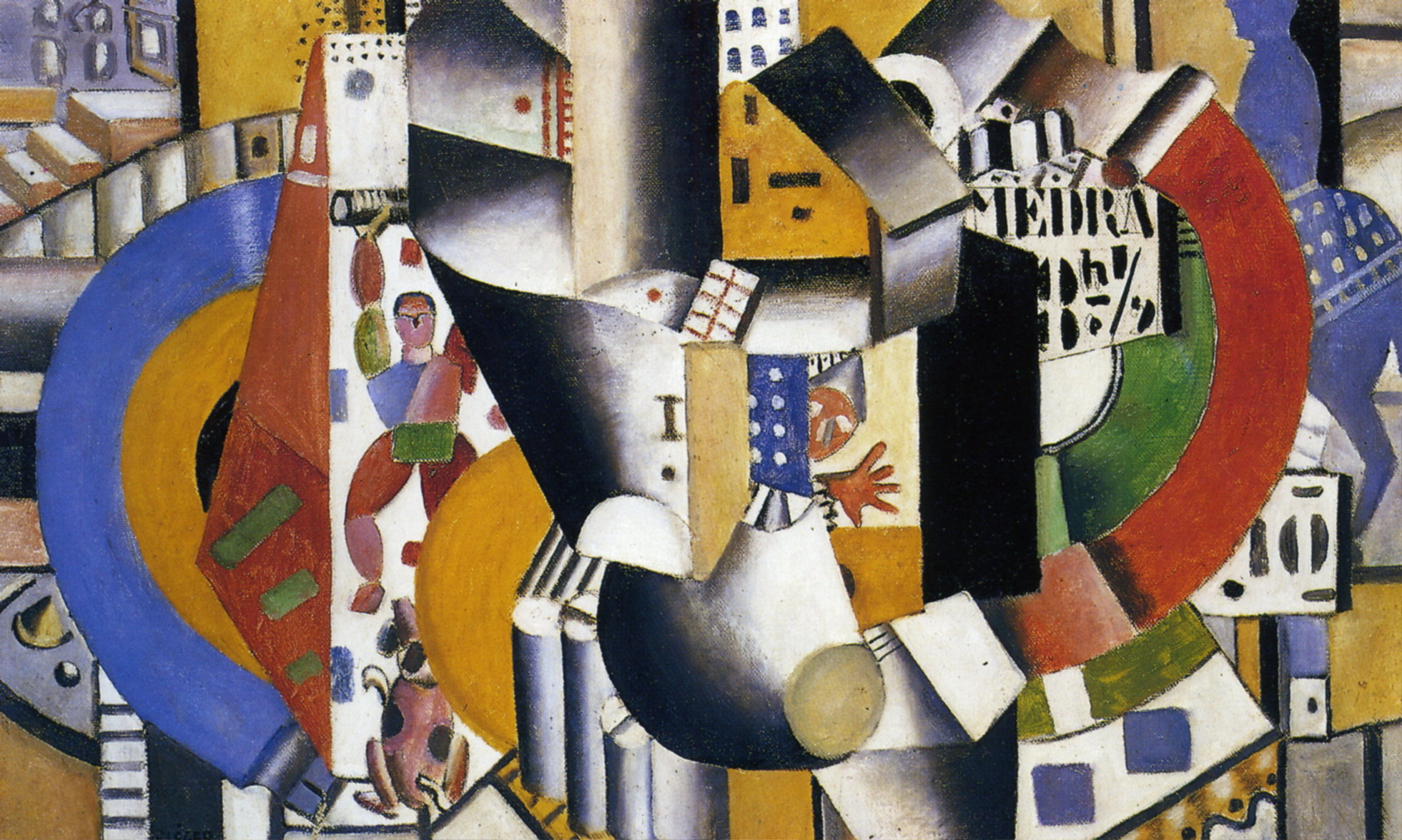This painting is a vibrant and chaotic blend of abstract and Impressionist styles depicting a bustling village scene. Dominating the composition are various shapes and colors, including circles, triangles, rectangles, and irregular forms in shades of blue, red, yellow, green, white, and black.

Key features include multiple flights of stairs—some brown and white—spanning the image, and diverse structures such as tall apartment buildings and houses hanging from a steel-colored fat pipe. In the lower section, a person, possibly a bodybuilder, is lifting weights within a white rectangle, colored in red, pink, blue, and yellow. Nearby, a dog sits calmly.

A partial image of a blue man riding a horse is visible, though only the back half of the horse and part of the rider can be seen. Amid the visual chaos, there are letters spelling out the word "Medra" along with numbers—an "8" and the fraction "1/9th." Additional features include blue domino-like pieces, an intricate mix of arcs in blue and red, and smaller details like a blue circle, a button, and several triangles, adding to the complex and dynamic nature of the painting.